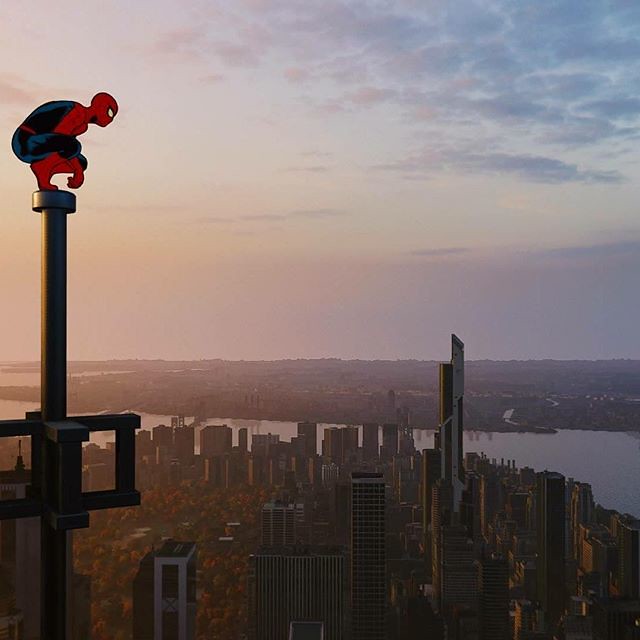The image captures a dramatic moment from a Spider-Man comic book movie, set against the backdrop of a cityscape at either dusk or dawn. The sky is painted in hues of blue, pink, purple, and orange with a few clouds scattered around, adding to the serene yet melancholic atmosphere. Below, a sprawling city stretches with tall skyscrapers and large buildings, possibly representing New York, though no iconic structures like the Chrysler Building or the Empire State Building are clearly identifiable. A river meanders through the cityscape, crossed by a distinctive bridge. Dominant in the foreground is a tall pole situated towards the left side of the image, characterized by four rectangular shapes midway up. Atop this pole, Spider-Man is crouched in his iconic red and blue costume, with the city unfolding beneath him. His intense gaze over the metropolis reflects his vigilant nature, heightened by the precision of the computer-generated imagery that brings him to life.